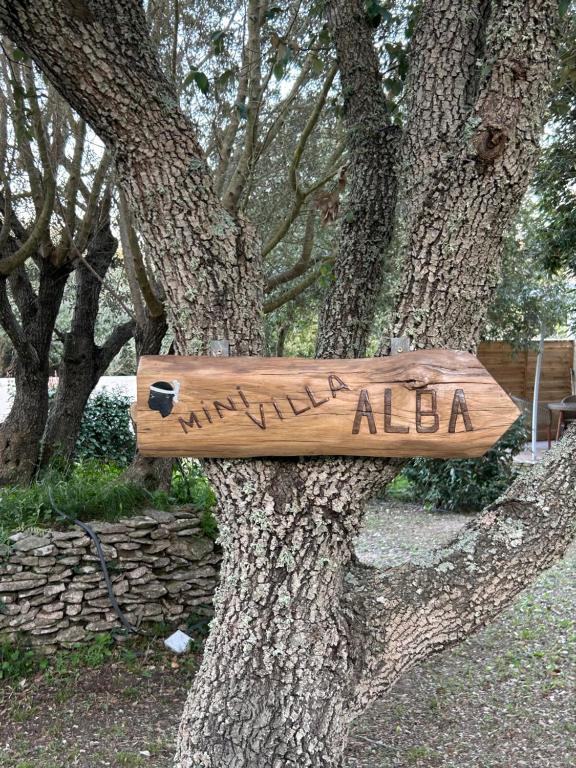This outdoor photograph captures a tree in portrait orientation, making the image taller than it is wide. The tree, centrally located, features rough, irregular gray bark and is scattered with about 10% light green moss climbing its trunk and main branches. Affixed to the tree is a light brown wooden arrow-shaped sign pointing to the right. The sign prominently displays the words "Mini Villa ALBA," with "ALBA" in capital letters and slightly darker. On the left side of the sign, there is an image of a dark-skinned face wearing a white headband, depicted in black paint.

The scene takes place in a wooded grove, suggesting a camping or open outdoor area. The background reveals additional trees with sparse foliage and various natural ground elements such as pebbles, weeds, and leaves. To the left, a stack of stones forms a retaining wall about a meter high, with some plants growing on top. Further details include a hint of a wooden fence on the right side, and a patio containing a brown table set is also faintly visible in the distance. The photograph was taken during the daytime, as indicated by the overall lighting and shadows present in the image.